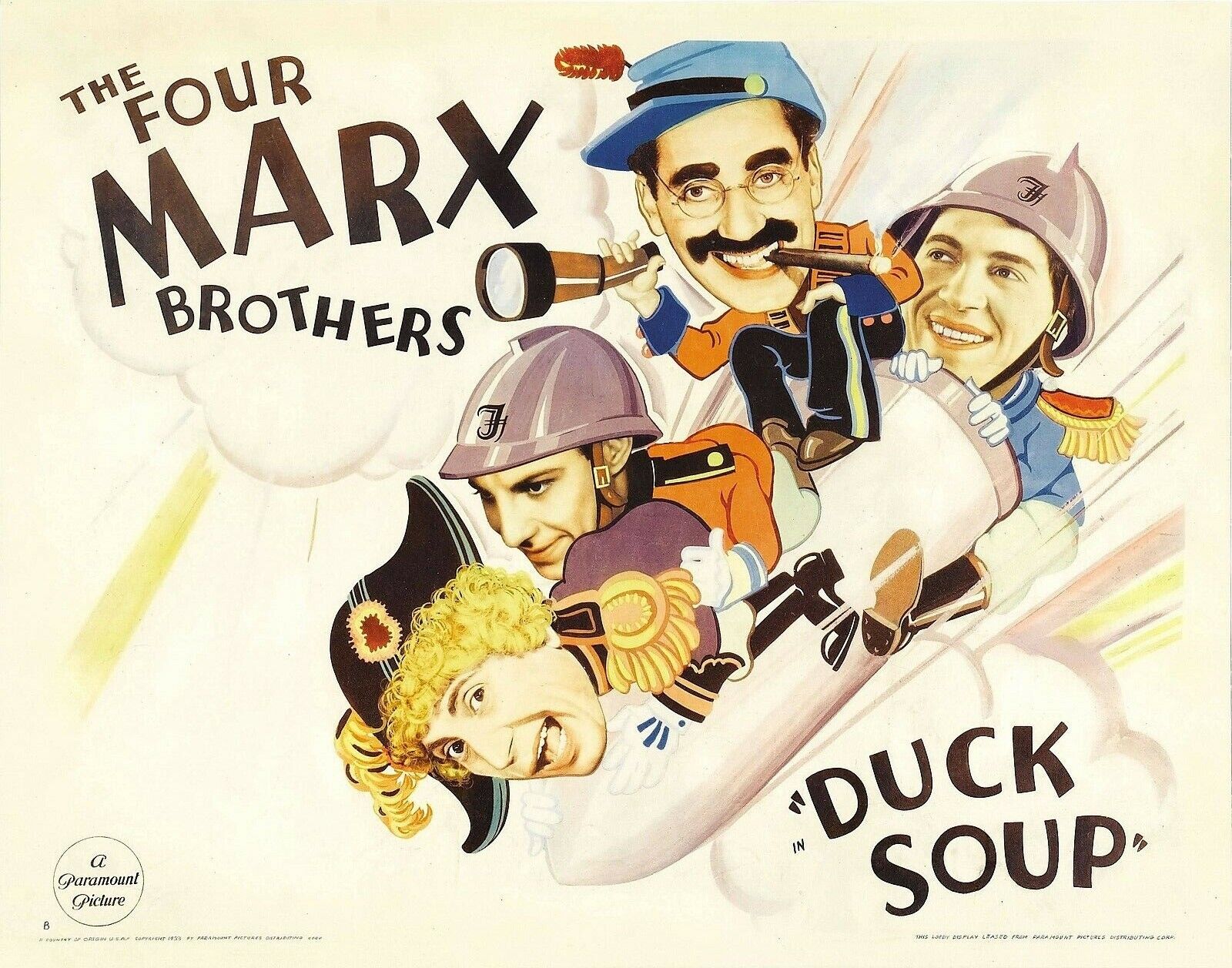An advertisement for the classic Marx Brothers movie "Duck Soup," presented as a whimsical colored-pencil illustration. The image features the four Marx Brothers cartoonishly depicted with exaggerated bodies in military attire, mounting a large rocket ship amidst a backdrop of explosions. Their faces are realistically portrayed, likely based on actual photographs or portrait paintings, blended with cartoonized elements. Groucho, recognizable by his signature mustache, glasses, and cigar, holds a telescope like a pirate's spyglass. Harpo, with his wild blonde curly hair, wears a pirate hat and clings to the rocket’s front. Another brother, donning a military helmet labeled with 'J,' clutches the back, while the fourth, dressed in a jockey-like outfit, straddles the midsection. The text “The Four Marx Brothers” appears in a puffy cloud above them, with “Duck Soup” similarly displayed below, and the Paramount Pictures logo is visible at the bottom left. This lively scene captures the zany spirit of the Marx Brothers and hints at the comedic chaos of the movie.